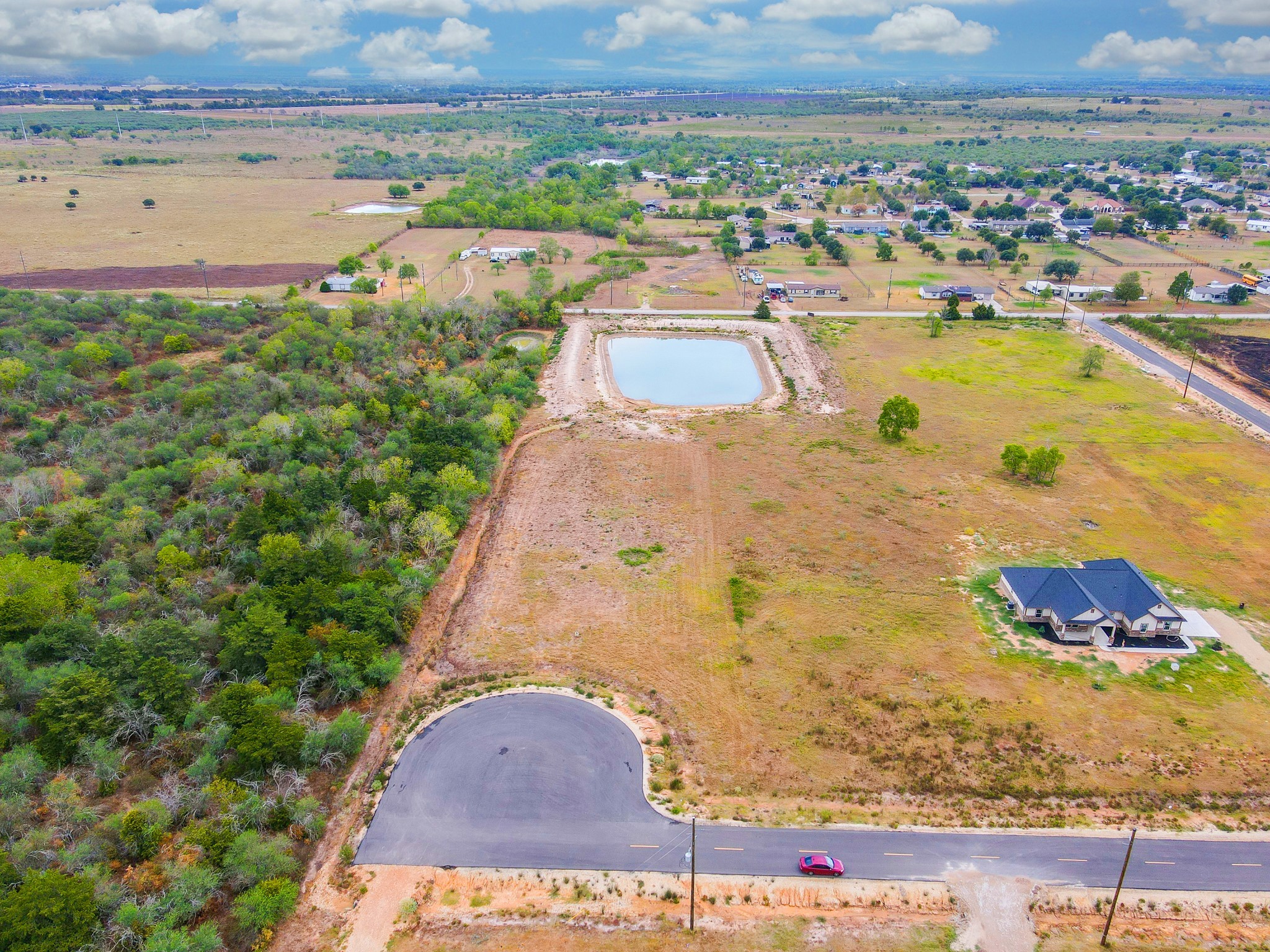An aerial photograph of Creekmore Meadows, Texas, depicts an expansive flat terrain characterized by varied land uses, both developed and undeveloped. Dominating the foreground is a sizable white house with a black-tiled roof and a partial view of its driveway to the right, adjacent to a cul-de-sac with a red car parked near a large turnaround. This dead-end road appears to be the entrance to the surrounding acreage designated for real estate development. To the left, a substantial forested area teems with green trees and shrubs, transitioning into a stretch of dry, yellow grassy land. A prominent feature is a large holding pond near the center of the image, encircled by a sand barrier. The landscape extends into a suburban setting with new homes and structures dotting the horizon, interspersed with fields and additional forested patches. Further back, flat green terrain stretches out to meet a distant line of small hills under a partly cloudy, blue sky.